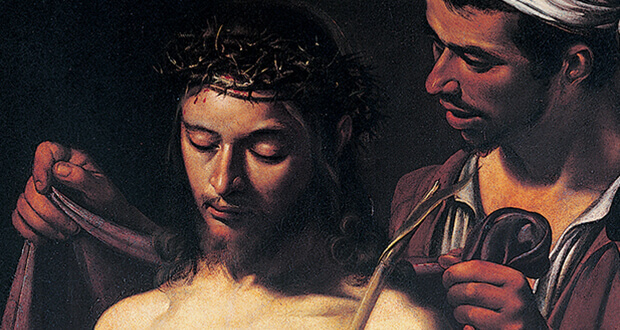This rectangular painting, with a black backdrop, is a poignant depiction of Jesus Christ at its center. Shirtless, Jesus is seen with a crown of thorns on his head, causing trickles of blood to flow down his forehead. His eyes are closed, and he has a scraggly brown beard and long brown hair. Clutched in his hand is a broken reed stick. Positioned to Jesus' right in the upper corner, a bearded man with a white turban and a red coat is wrapping a robe around Jesus' shoulders. The man appears to be speaking to Jesus, his mouth slightly open and his gaze directed at Jesus, who is looking downward. The composition effectively highlights the contrast between the two figures and the somber, dark background emphasizes the solemn mood of the scene.